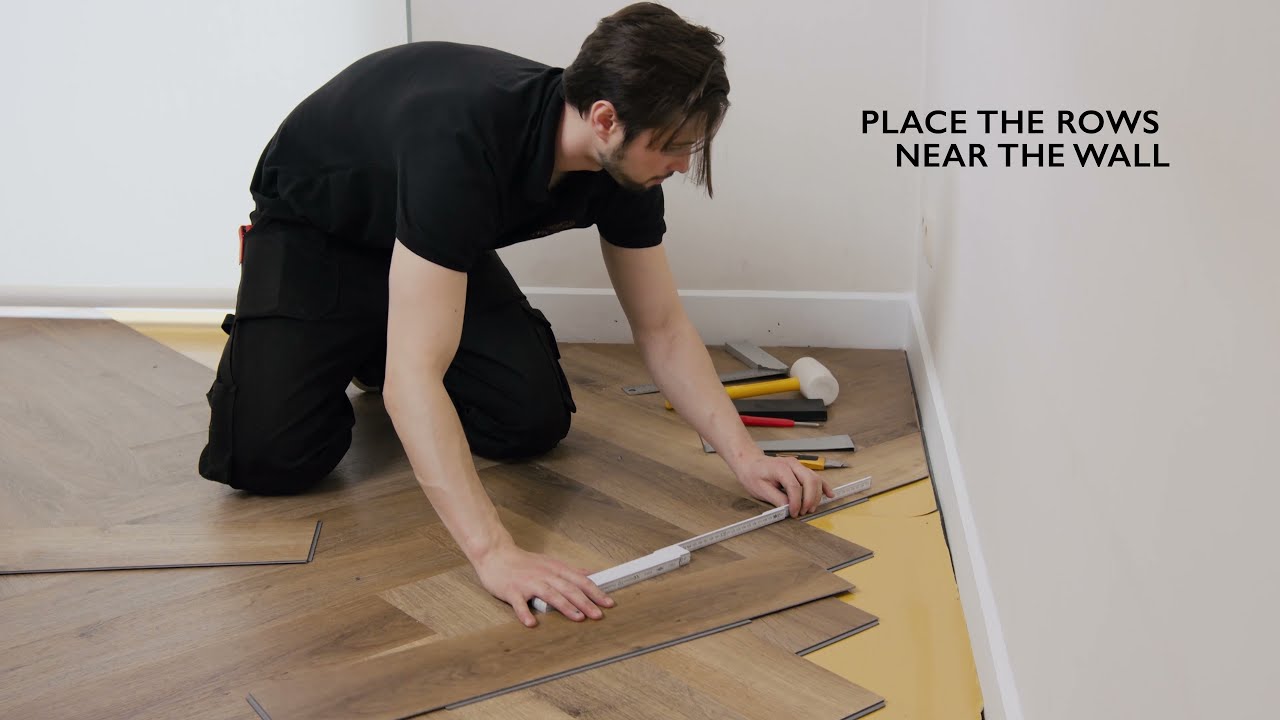The image depicts a detailed step-by-step tutorial on how to lay laminate flooring as a do-it-yourself project. At the center of the photograph is a man dressed in black pants and a black shirt, kneeling on a partially installed medium brown, wood-look laminate floor with lighter brown accents. He appears to be measuring a piece of laminate with a folding ruler or angle measuring device to fit it precisely against the wall behind him, which is white with an even whiter crown molding. Surrounding him are various tools including a white and yellow-handled rubber mallet, a level, and several rulers. To his left, a few more laminate pieces are ready to be installed. Towards the top right of the image, black bold text instructs, "place the rows near the wall." This setup indicates a thorough and detailed approach to DIY laminate flooring installation.